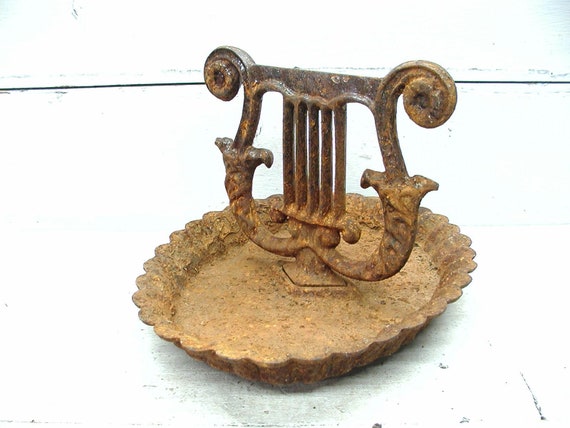The photograph showcases an antique cast-iron boot scraper, resting on an ornate, pie-shell-like bowl with a ruffled ridge. Both objects, possibly made of bronze, exhibit significant wear with visible rust and dirt. The boot scraper, positioned in the center, features a distinctive arch at the bottom flanked by five bars and is adorned on each side with elegant, swirling patterns reminiscent of cinnamon rolls. The scene is brightly lit against a white surface and background, casting a noticeable shadow from the object. The detailed craftsmanship suggests an air of elegance, though the condition implies it is quite aged and neglected.